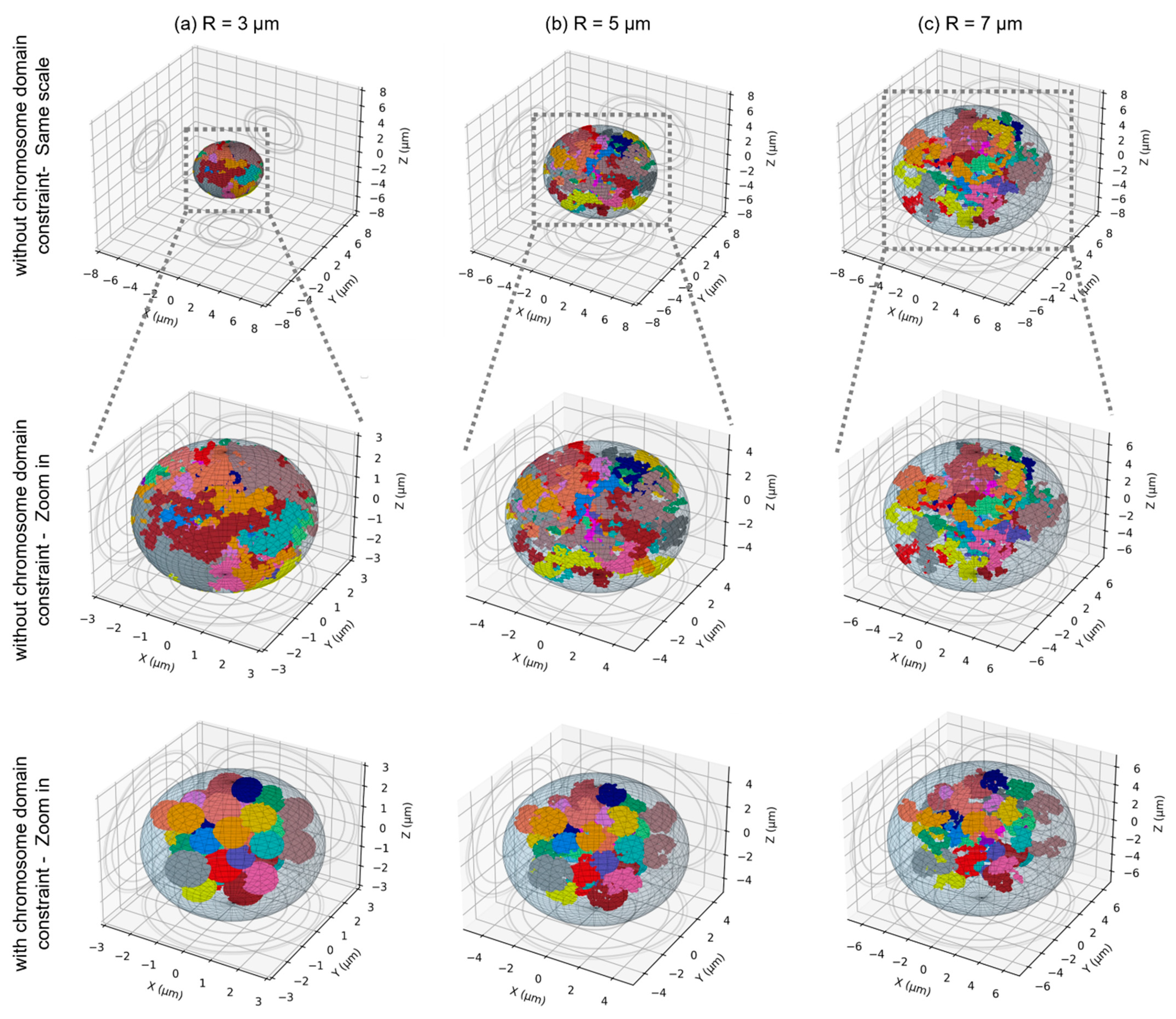This image showcases nine scientific diagrams arranged in a three-by-three grid, organized into three columns and three rows. Each diagram represents a three-dimensional grid, marked with x, y, and z-axes. The columns are labeled at the top as follows: "A, R = 3 micrometers," "B, R = 5 micrometers," and "C, R = 7 micrometers." The rows, from top to bottom, are labeled: "Without Chromosome Domain Constraint, Same Scale," "Without Chromosome Domain Constraint, Zoom In," and "With Chromosome Domain Constraint, Zoom In."

The first row displays the most zoomed-out images, maintaining a constant scale. The second row features medium zoomed-in versions of the same diagrams, with clear zoom lines connecting to the corresponding images in the first row. The third row presents the most zoomed-in images, all of which include chromosome domain constraints and exhibit no zoom lines from the second row. Each diagram centers on an oval shape filled with various colored, blob-like patterns, which may represent biological or scientific elements such as microbes or puzzle pieces. The axes are scaled differently for each row to accommodate the level of zoom and detail: the top row ranges from -8 to 8, the middle row ranges from around -3 to 4 or -6 to 6, and the bottom row similarly ranges from -3, 4, and 6 to their positive counterparts.